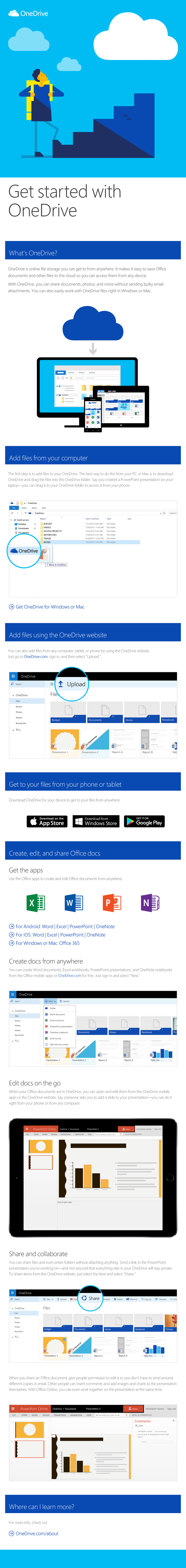A blurry screenshot featuring a long vertical layout with a short horizontal span. At the top, a blue header displays a trio of clouds—one white and two light blue. Below, a simplistic stick figure wearing a yellow jacket ascends a staircase where the first three steps are black, transitioning to blue steps higher up. A phrase underneath reads "Get started with OneDrive."

Following this, a wide blue bar stretches across the image, adorned with unreadable white text. Beneath this bar, a white background appears with black text alongside a blue cloud graphic, which includes arrows pointing towards a computer, a phone, and a tablet. Another blue bar with obscured white text lies below. Additional sections show black text on a white background accompanied by dropdown menus from a program interface, succeeded by another blue bar.

Moving further down, the image contains three black bars followed by colored boxes in green, blue, red, and purple, alongside more dropdowns. To the side, a profile view of a cell phone is noticeable among various textual elements and dropdown menus, concluding with a blue bar and a lighter blue bar at the image's bottom.